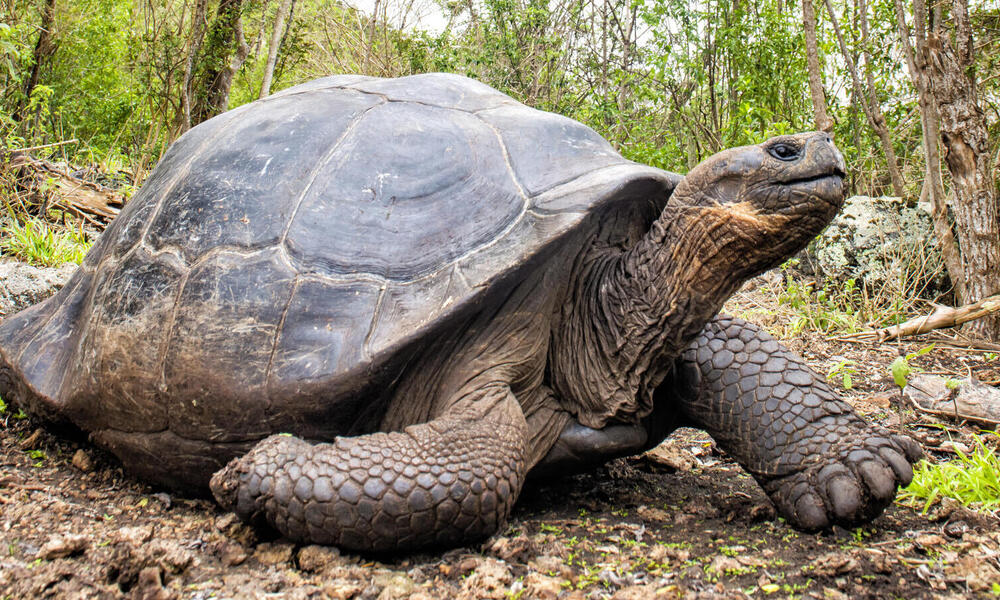This high-definition, wide-angled photograph showcases a large turtle, possibly a giant one, ambling slowly across a dirt and gravel path in a wooded area. The turtle's leathery, veiny neck, showing signs of age with light brown patches, is extended towards the upper right corner of the image. Its front legs are stretched forward, revealing clawed feet with a diamond-shaped pattern. Though its hind legs remain unseen, the shell—black and tattered with intricate lines—rests solidly on the ground. Surrounding the turtle are tree trunks, green leaves, dried foliage, and old branches, grounding it firmly within the forest setting. This close-up captures both the turtle's detailed textures and the natural woodland backdrop.